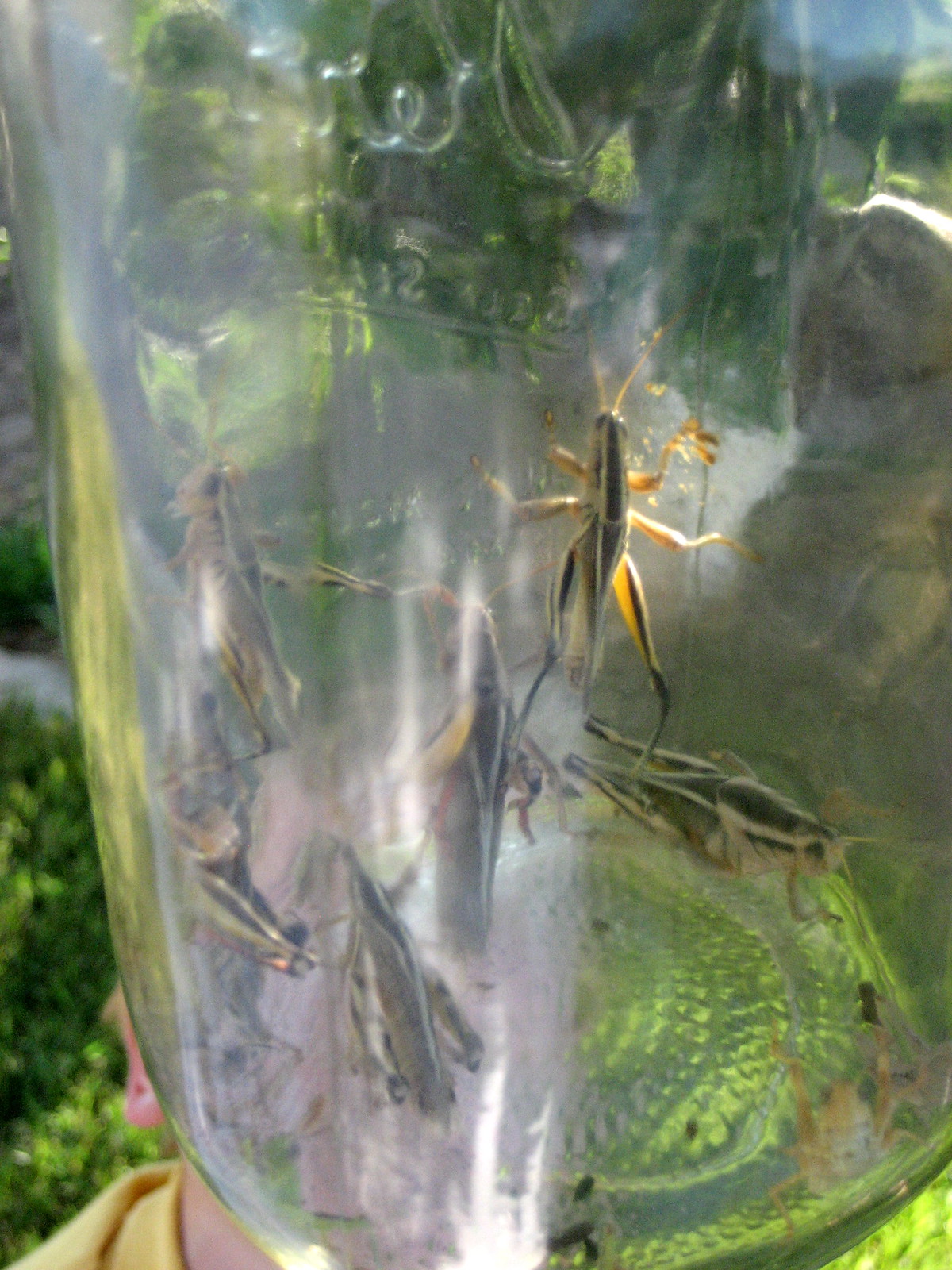The photograph captures a vibrant outdoor scene featuring a glass mason jar filled with approximately eight grasshoppers and crickets, exhibiting yellow, green, and black coloration. The jar is held up by a child, with the lower part of the image showing a glimpse of the child's yellow shirt and ear, while their face remains obscured. Sunlight filters through the glass, casting reflections that partially obscure the insects within. In the background, there is lush green grass and foliage from bushes, adding to the natural setting. The insects are in various positions—some spread-eagle on the jar walls, others perched or crawling on the jar's floor. The sunlight illuminates their bodies, making their translucent limbs almost glow.